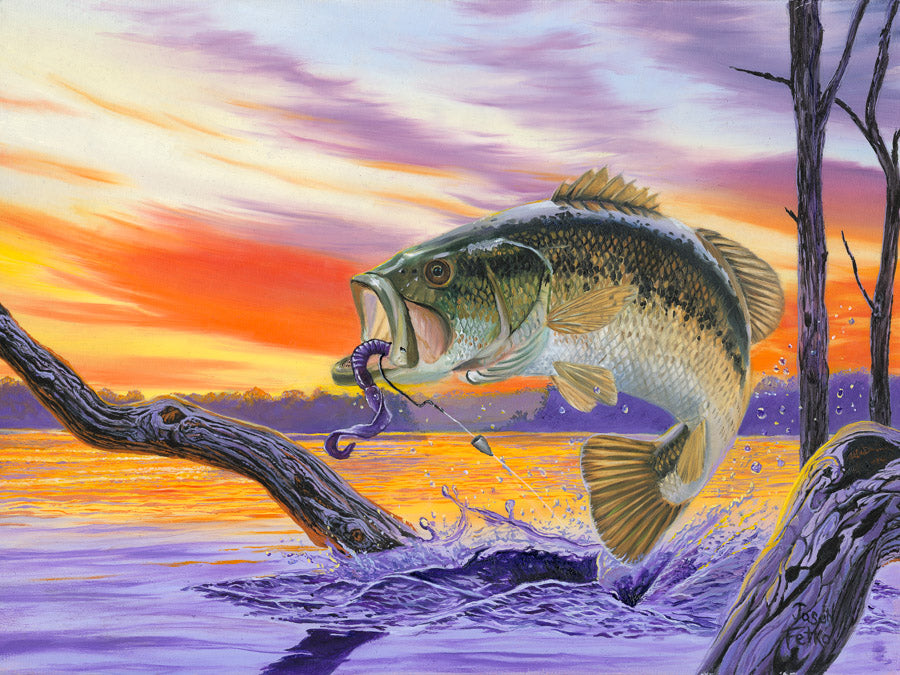This detailed and vibrant painting captures a dramatic scene of a fish leaping out of purple waters at sunset, ensnared by a fishing hook. The fish, resembling a bass, features an army green top with a dark black-brown gradient and a gleaming silver underside. Its scales glisten, complemented by gold hues on its tail and fins. The fishing hook is prominently lodged in the fish's mouth, with a compelling purple worm attached that likely lured the fish. The fish's body forms a distinctive C shape, with its tail bent at a sharp 90-degree angle, conveying a sense of its struggle. 

The backdrop unveils a mesmerizing sky painted in vertical streaks of purple, orange, yellow, cream, and white, adding depth to the sunset. Purple clouds blend into orange hues near the horizon, enhancing the scene's whimsical atmosphere. Emerging from the water, three prominent tree branches devoid of leaves extend upwards, two on the right and one on the left, immersed in the purple reflection of the water that shifts to orangey tones farther back. In the distant horizon, a row of purple trees lines the scene. The composition is signed "Jaskut Forte" at the bottom right, adding an element of authenticity. Altogether, the painting brilliantly captures the raw emotion and vivid colors of a lively sunset fishing scene.